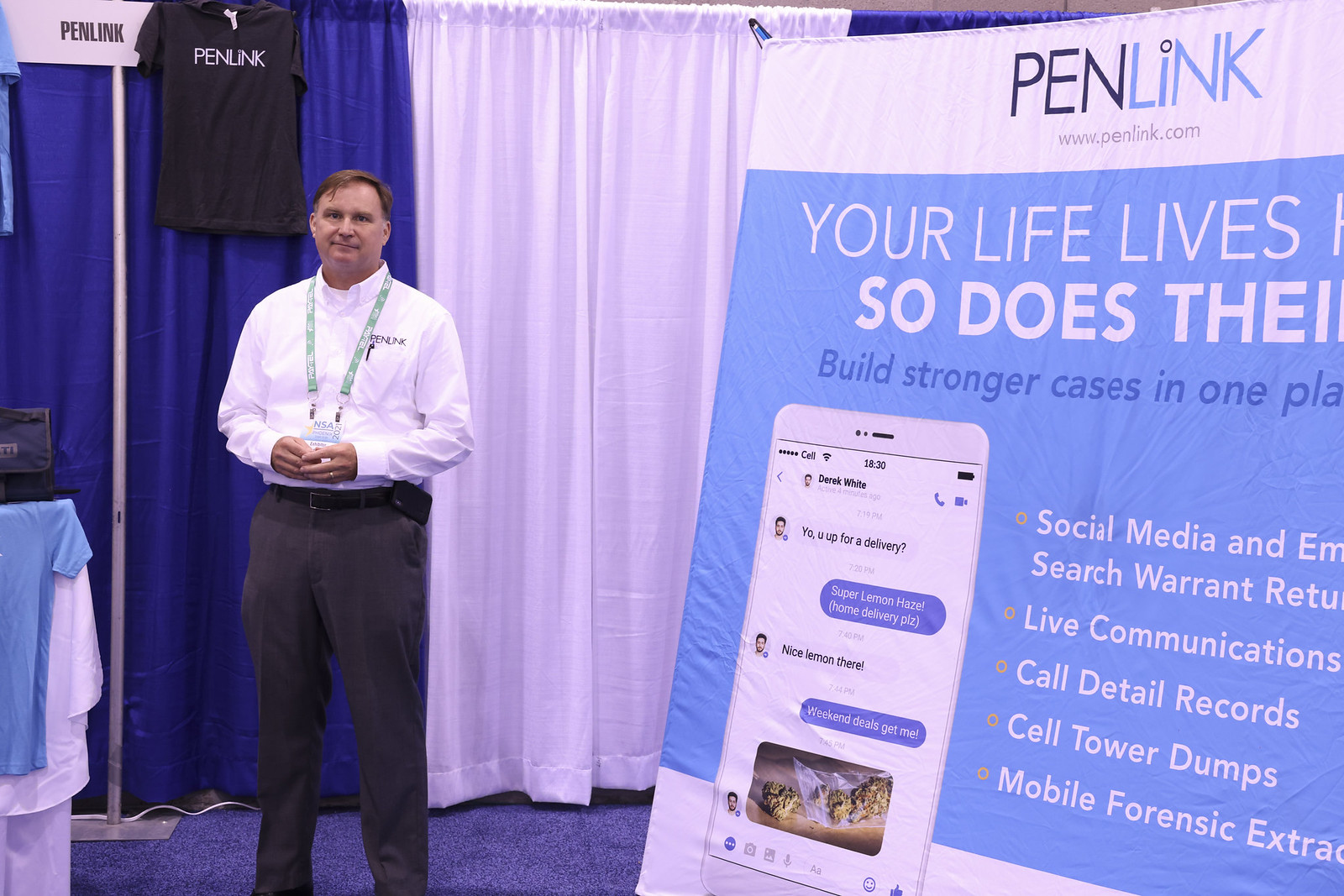The image captures a man at a booth within a conference or trade show, likely the NSA 2021 event. The man, dressed in a white button-down shirt emblazoned with the logo "PenLink" just above the left pocket and dark grey pants, stands facing the camera. He wears a green lanyard with a badge around his neck. To his left hangs a black t-shirt with the "PenLink" logo, and behind him are blue and white curtains, likely serving as dividers for other booths. Dominating the right side of the image is a large sign that also reads "PenLink" at the top, featuring a mock-up of a phone displaying a Facebook Messenger conversation about a delivery. The poster showcasing "PenLink" provides a partial but critical view of its services, emphasizing capabilities in building stronger cases by consolidating social media, search warrant returns, live communications, call detail records, and cell tower dumps, among other forensic data. The entire scene suggests a professional setup aimed at promoting PenLink's specialized tools for law enforcement and investigative purposes. The colors in the setting range from light blue and dark blue to white, black, and various shades of grey, creating a corporate ambiance for the expo environment.